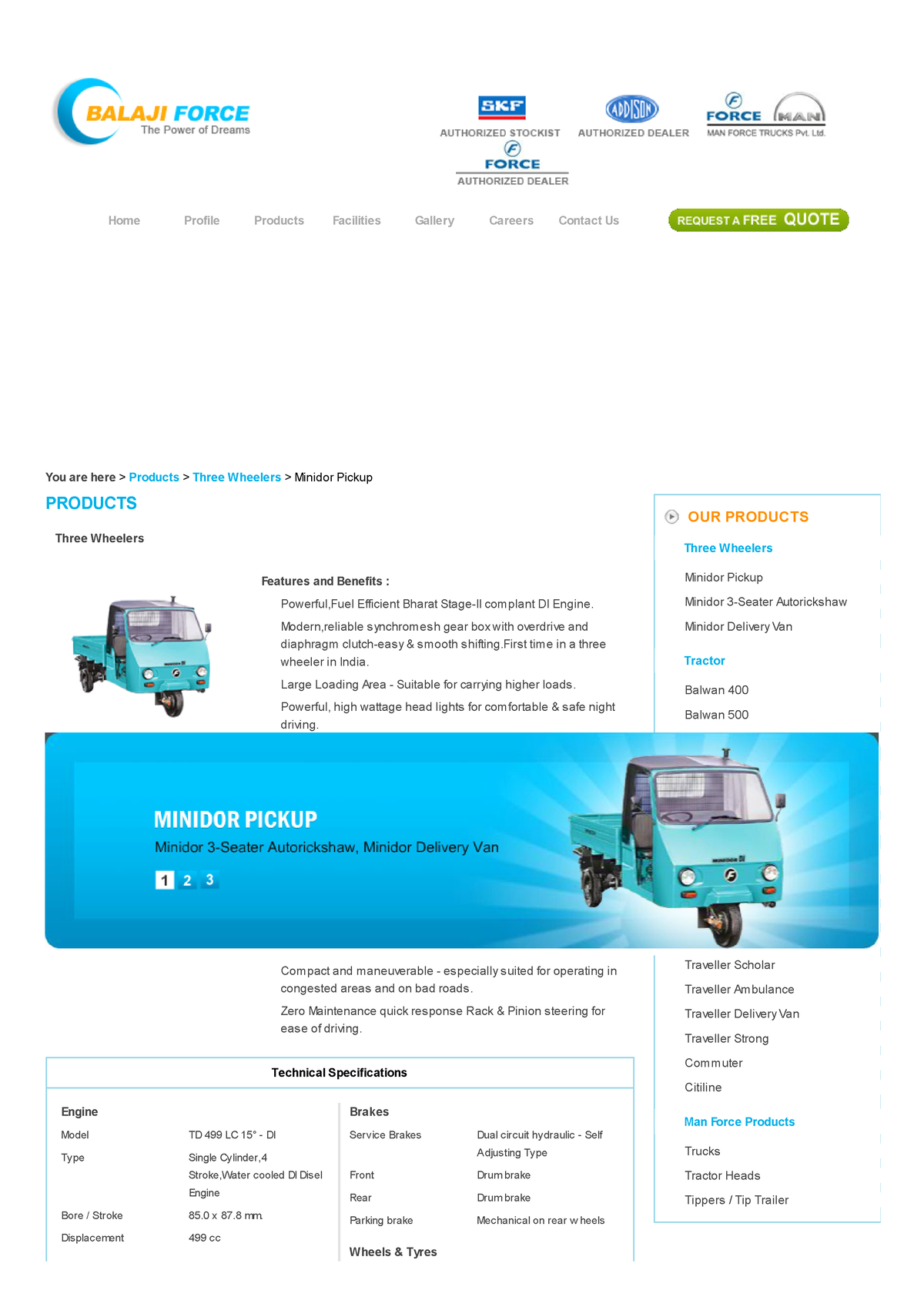**Descriptive Caption for Mini-Door Pickup Product Page**

The product page for the Mini-Door Pickup, a versatile three-seater auto rickshaw, details both the Mini-Door delivery van and passenger auto rickshaw models. Central to the page is a visually striking, two-tone blue box, with a darker blue outer border and a lighter blue inner section. Inside this box is an image of the rickshaw itself, showcasing key features: an automatic cab, a motor, and distinctive lighting. The rickshaw has dual circular white headlights positioned above two rectangular red reflecting lights, with a brand icon housed in a black circle centrally placed between the headlights. The cab, reminiscent of a small truck or golf cart, displays a visible steering wheel through its rectangular windshield. This three-wheeled vehicle has a single front wheel and two rear wheels, with the rear right wheel visible in the image. The open-bed design at the back resembles a mini pickup truck, ideal for light cargo.

Surrounding the image is an ethereal light blue and white accent, mimicking the effect of glowing rays or sunlight. Below this central image, the page is text-heavy, beginning with navigational breadcrumbs: "You are here" followed by arrows linking to "Products," then "Three Wheelers," and finally "Mini-Door Pickup."

The product page further features another image of the rickshaw, supplemented by detailed descriptions of its features and benefits. Technical specifications are methodically outlined in a box at the bottom, comprising two main columns, each with two sub-columns. These cover various aspects like the engine, brakes, and wheel types. On the right side, a navigation bar includes several product categories in orange text, labeled "Our Products," followed by sub-categories such as "Three Wheelers," "Tractors," and "Man Force Products," each with specific product names listed in black under blue subheadings.